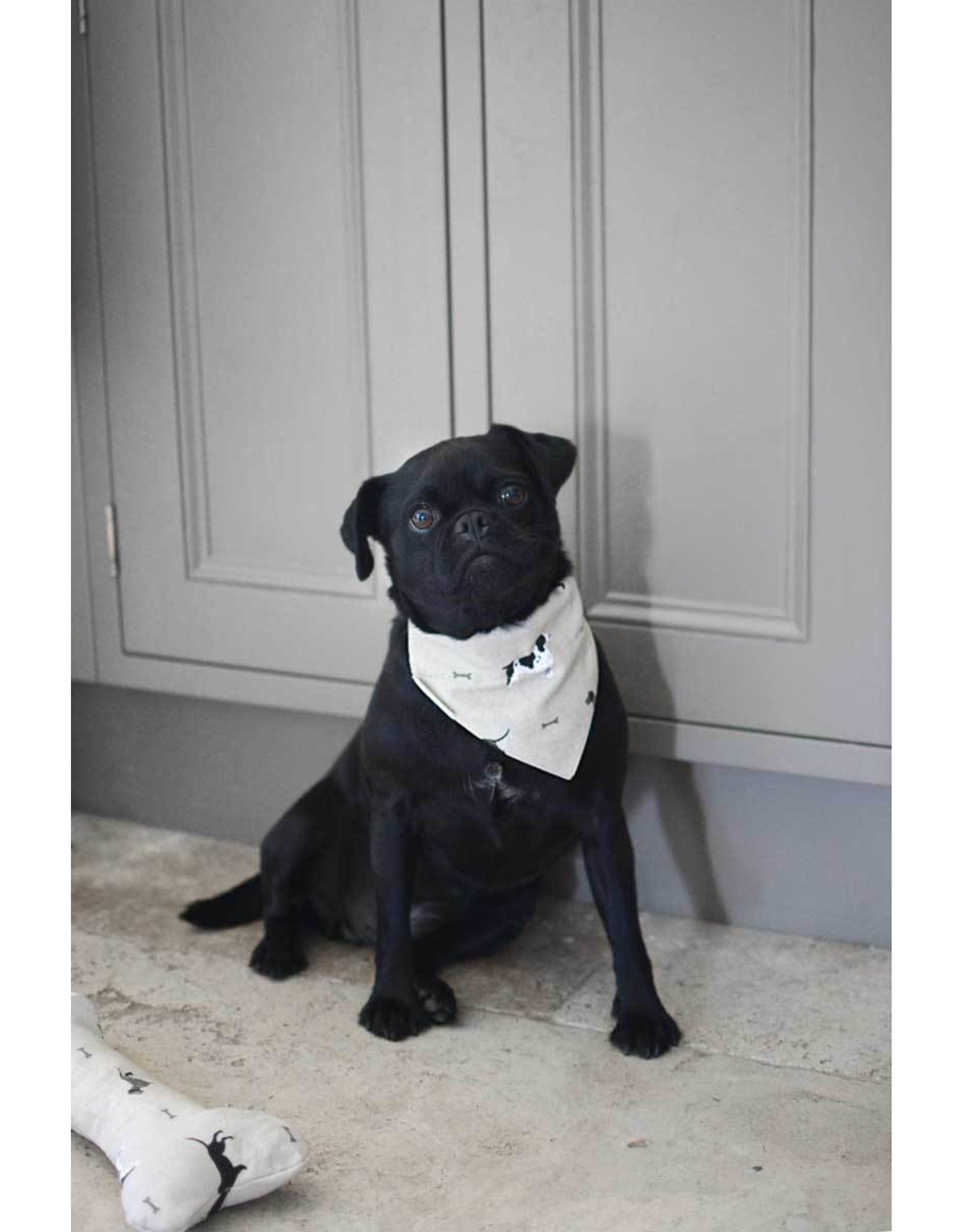In the image, there is a photograph of a small black puppy sitting on white, flat concrete flooring. The puppy, situated almost at the center of the image, is wearing a light grayish-tan handkerchief adorned with tiny bone and dog prints around its neck. To the bottom left of the dog, there is a bone-shaped stuffed toy featuring the same pattern of bones and dogs as the handkerchief. The background shows a white panel cabinet door with hinges, giving the scene an indoor setting. The dog's posture is a seated position, looking directly at the viewer. The detailed prints on both the handkerchief and stuffed toy create a cohesive visual theme.